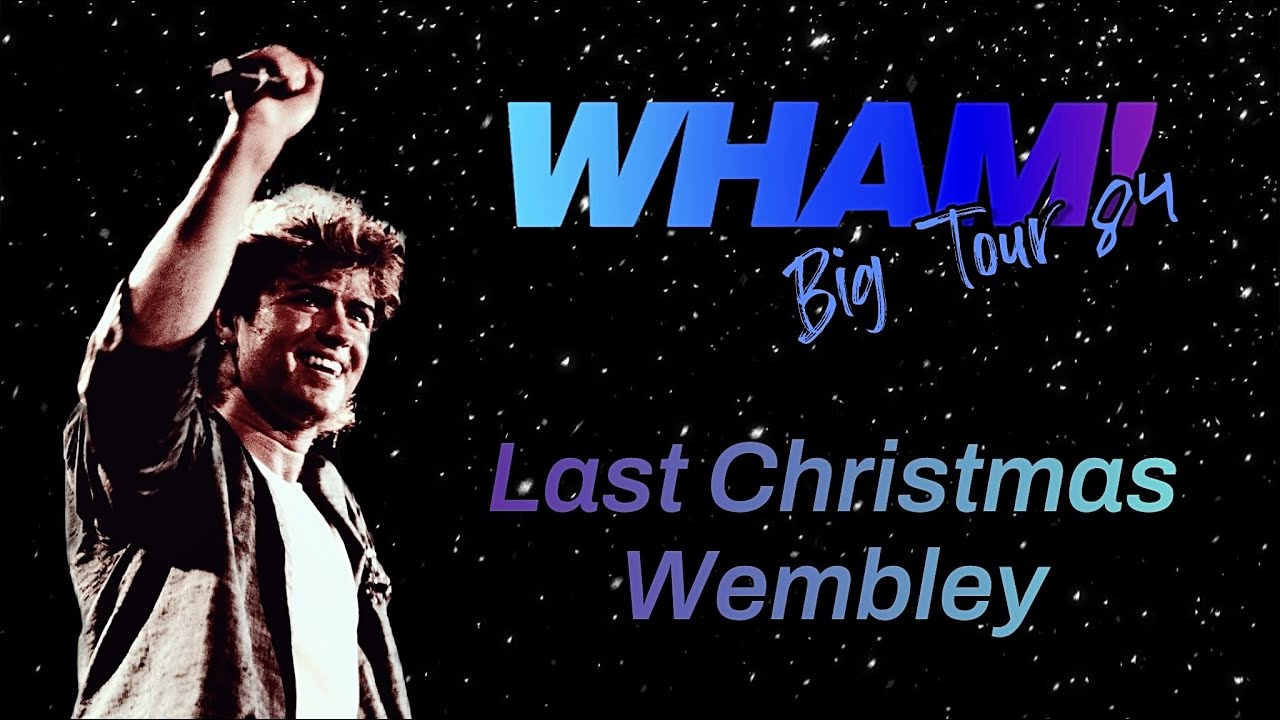This poster advertises a concert tour by the band Wham! The background is predominantly black, dotted with white specks resembling stars, creating a starry night effect. At the top right, prominently displayed, is the name "Wham!" written in a gradient of blue to purple, with an exclamation point in purple. Below this, the text "Big Tour 84" is overlaid in bold letters. Further down, "Last Christmas Wembley" is also highlighted, featuring a color gradient from purple to light blue. On the left side of the poster, there is an image of a young George Michael. He is smiling and holding a microphone above his head with his right hand. His hair is feathered and styled in a brownish mullet. He wears a white t-shirt under a gray button-down shirt that is open, with the sleeves casually rolled up. The overall design and imagery evoke the vibrant and youthful energy of the early 1980s.